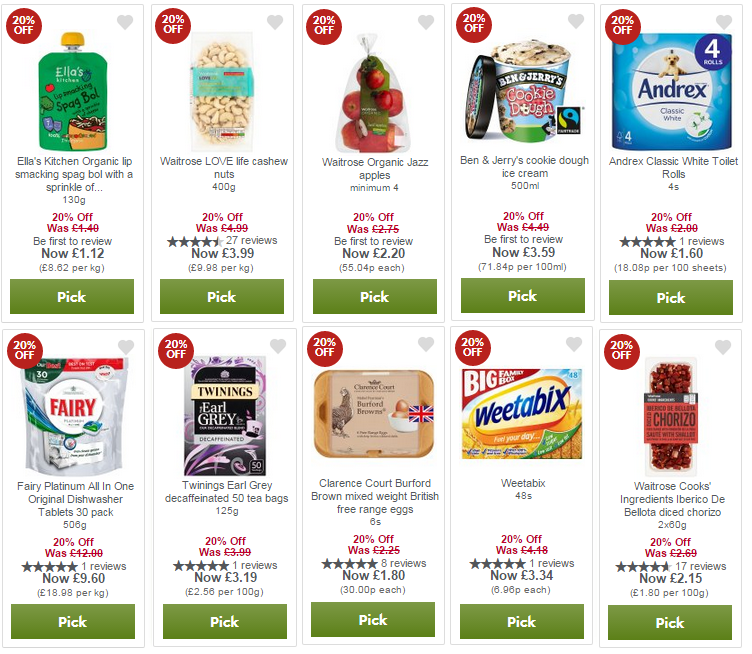This image showcases a coupon section within a grocery store shopping application, designed for users in the British Isles. The screen displays two rows, each containing five rectangular boxes, which are taller than they are wide. Each box features a product image at the upper center, and a prominent red circle with white text in the upper-left corner indicating a "20% off" discount. 

Below the image, there is a detailed description of the item, including the price difference. For example, "Waitrose Organic Jazz Apples, minimum 4, was £2.75, now £2.20." Another item listed is "Twinings Earl Grey Decaffeinated 50 Teabags." Additionally, "Waitrose Cooks' Ingredients Iberico De Diced Chorizo, 2 at 60 grams," is available. 

At the bottom of each box, a green rectangle marked "Pick" allows users to select the item. The discounted prices are indicated in pounds, emphasizing that this service is specific to the British Isles. Users can easily browse and select the items they want to purchase, making their online shopping experience convenient and efficient.